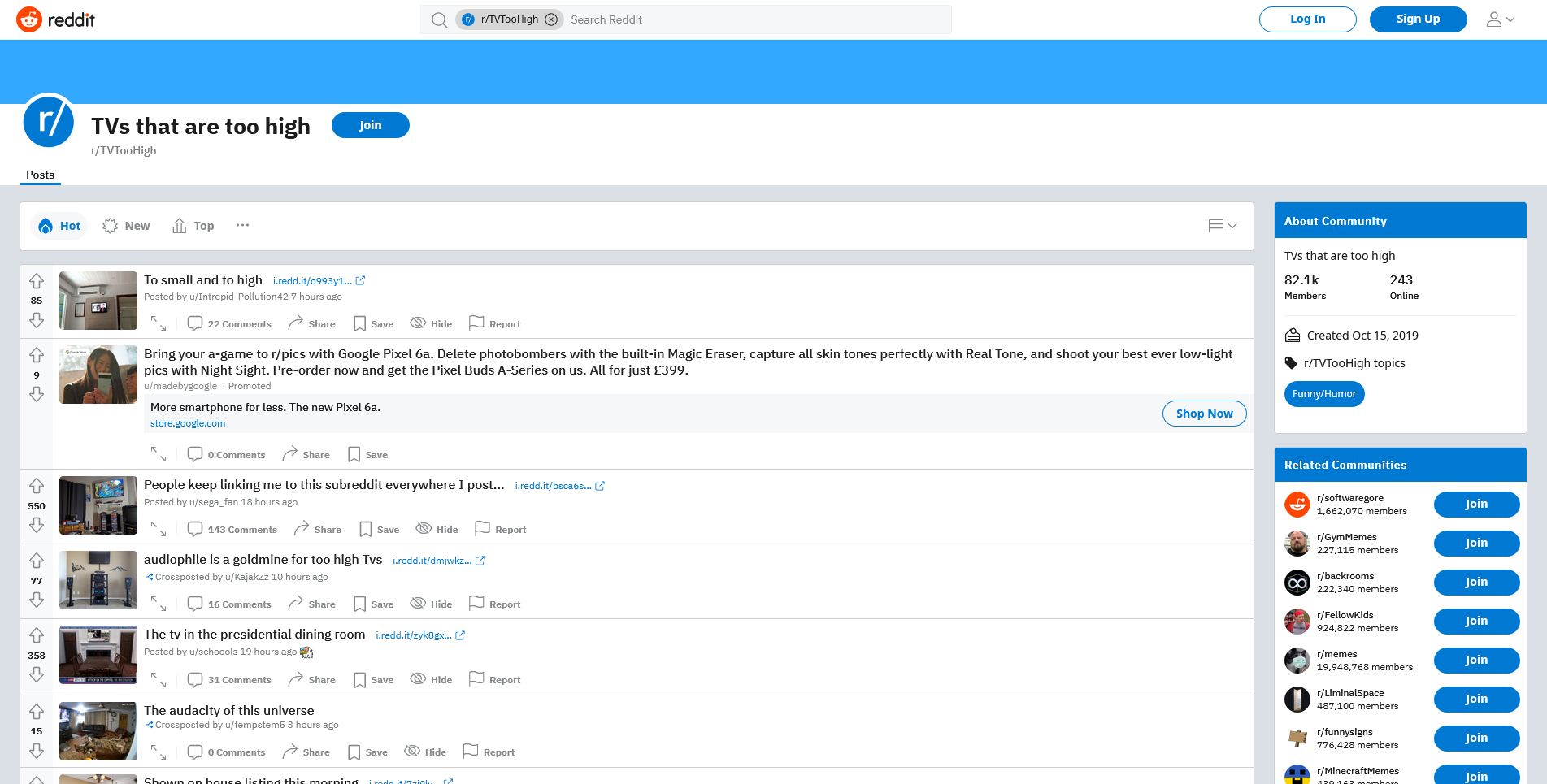This image showcases a webpage from the Reddit website. The text on the page is displayed in a very small font, making it difficult to read even when magnified. 

In the top left corner, the Reddit logo is prominently visible. Adjacent to the logo is the search bar, which allows users to search for content across Reddit. To the right of the search bar, there is a white, pill-shaped button labeled "Login," and next to it, a blue button that says "Sign Up" followed by an icon of a person.

Highlighted in blue on the page is the title of a subreddit, "TVs that are too high," along with a button that says "Click to join." Directly beneath this, there are options to filter posts by "Hot," "New," and "Top."

On the right side of the page, there is a clickable section related to the community. Below this section, there is a list of related communities. To the left, underneath the post sorting options, a few posts from the subreddit can be seen, but the small text makes them difficult to discern clearly.

The overall layout of the page includes standard elements typical of the Reddit interface, including navigation and community interaction features, but is hampered by low legibility when zoomed in.